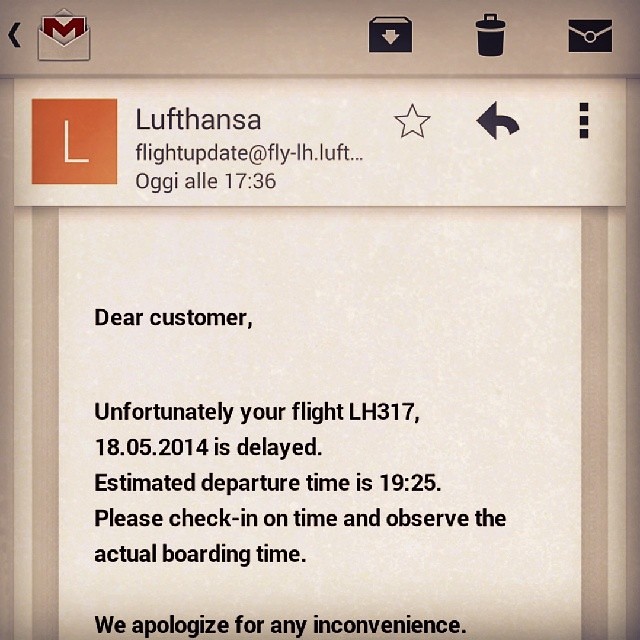This is a color photograph of a filtered screenshot, appearing to be from the Gmail app on a phone. The image shows an email from Lufthansa, the German airline, regarding a flight delay. At the top left, the old Google Mail logo (an M inside an envelope) is visible alongside icons for Inbox/Archive, Trash, and Check Mail on the top bar. The subject field contains "Lufthansa flight update at FLY-LH OVL 1736" with a white 'L' in an orange square. To the right of the subject are a star icon, a reply arrow, and a three-dot menu button. The email's body, displayed over a tannish background with black letters, reads: "Dear customer, unfortunately your flight LH317 on 18-05-2014 is delayed. Estimated departure time is 19:25 (military time). Please check in on time and observe the actual boarding time. We apologize for any inconvenience." The screen also features a gradient filter, darkening toward the edges.